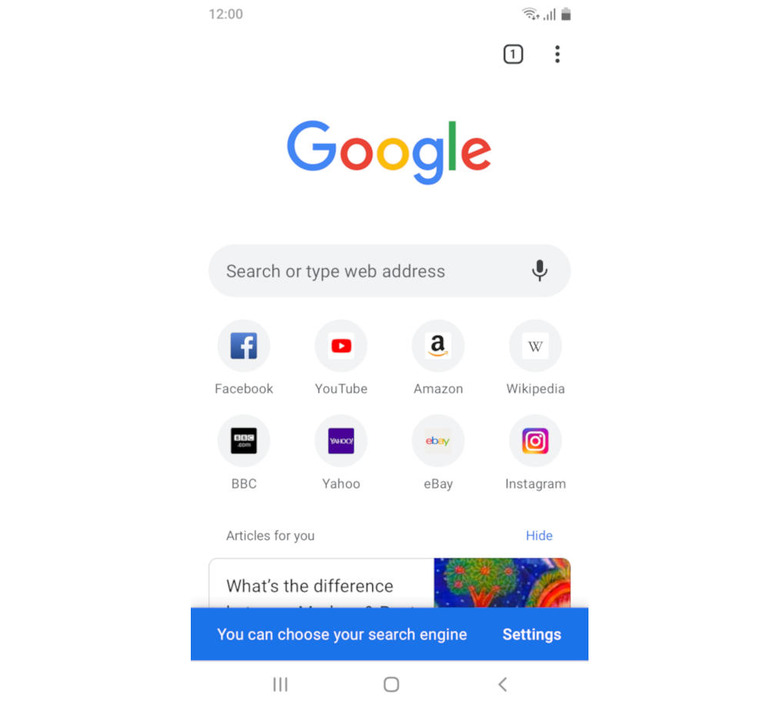A detailed and cleaned-up caption for the described image:

"This is a screenshot of a smartphone displaying a web browser interface. At the top, there is a blue rectangular banner with text indicating that you can choose your search engine and settings, specifically mentioning Google. The screen shows full signal strength and a fully charged battery icon. Below the blue banner, the search bar displays the Google logo with options to search by typing a web address or using the microphone. Popular website icons such as Facebook, YouTube, Amazon, Wikipedia, BBC, Yahoo, eBay, and Instagram are shown underneath the search bar, suggesting quick access to these sites. The phrase 'Articles for you' is displayed, indicating a personalized content section. The background appears white, adding a clean, minimalistic look to the interface. The time is shown as 12 o'clock. The overall layout suggests a user-friendly experience for browsing the web and accessing frequently used applications on a smartphone."